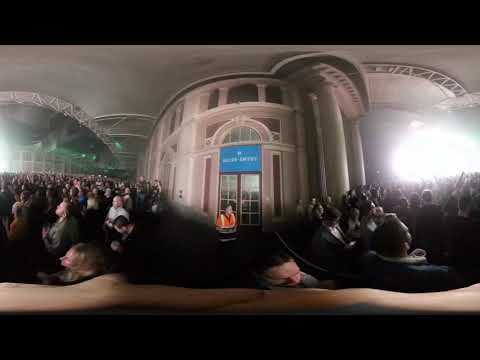This fisheye, landscape-oriented photograph, composed of three seamlessly blended images, captures a large, vibrant event. The top and bottom borders feature horizontal black bars that frame the scene. Central to the image are double doors with 12 panes of glass each and a blue sign with unreadable white text above them. In front of these doors stands a person in an orange safety vest, likely a security guard, greeting or directing attendees. 

To the left and right of this central scene, a vast audience fills the auditorium, their attention divided. On the left, people gaze towards a distant, somewhat greenish light, while those on the right side look towards a strikingly bright white light that dominates the background. The auditorium itself features a cream-colored or gray ceiling supported by circular columns, contributing to the grandeur of the venue. The overall distorted and abstract appearance gives the image a unique, almost surreal quality, likely achieved using a specialized fisheye filter.